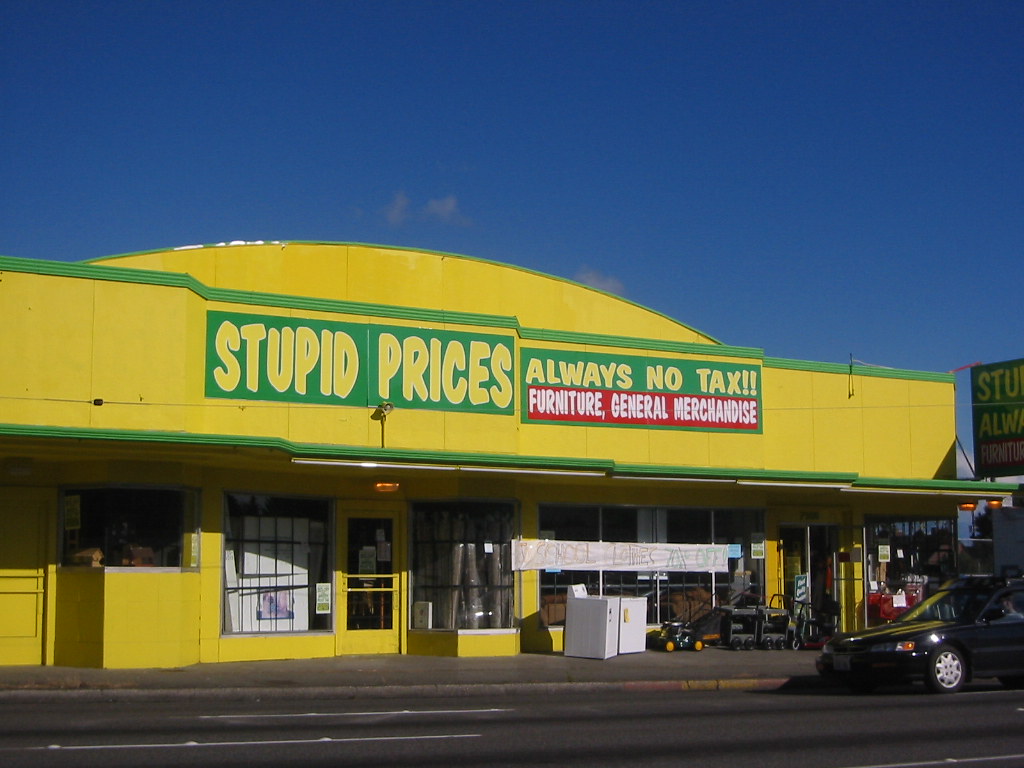This photograph captures a vibrant standalone store set against a clear blue sky. The entire storefront is painted a striking bright yellow, accented with vivid green trim. Prominently displayed in bold capital letters, the store's name, "STUPID PRICES," is easily visible. Adjacent to this sign, another sign reads "ALWAYS NO TAX" in yellow lettering on a green background. Below these, a red sign with white text announces "FURNITURE GENERAL MERCHANDISE." In front of the store, various items including a white washer and dryer, and a lawnmower are arranged, suggesting a diverse inventory. A black car is captured in motion as it drives by. Additionally, some signs in the windows highlight a promotional offer: "SCHOOL CLOTHES TAX OFF."